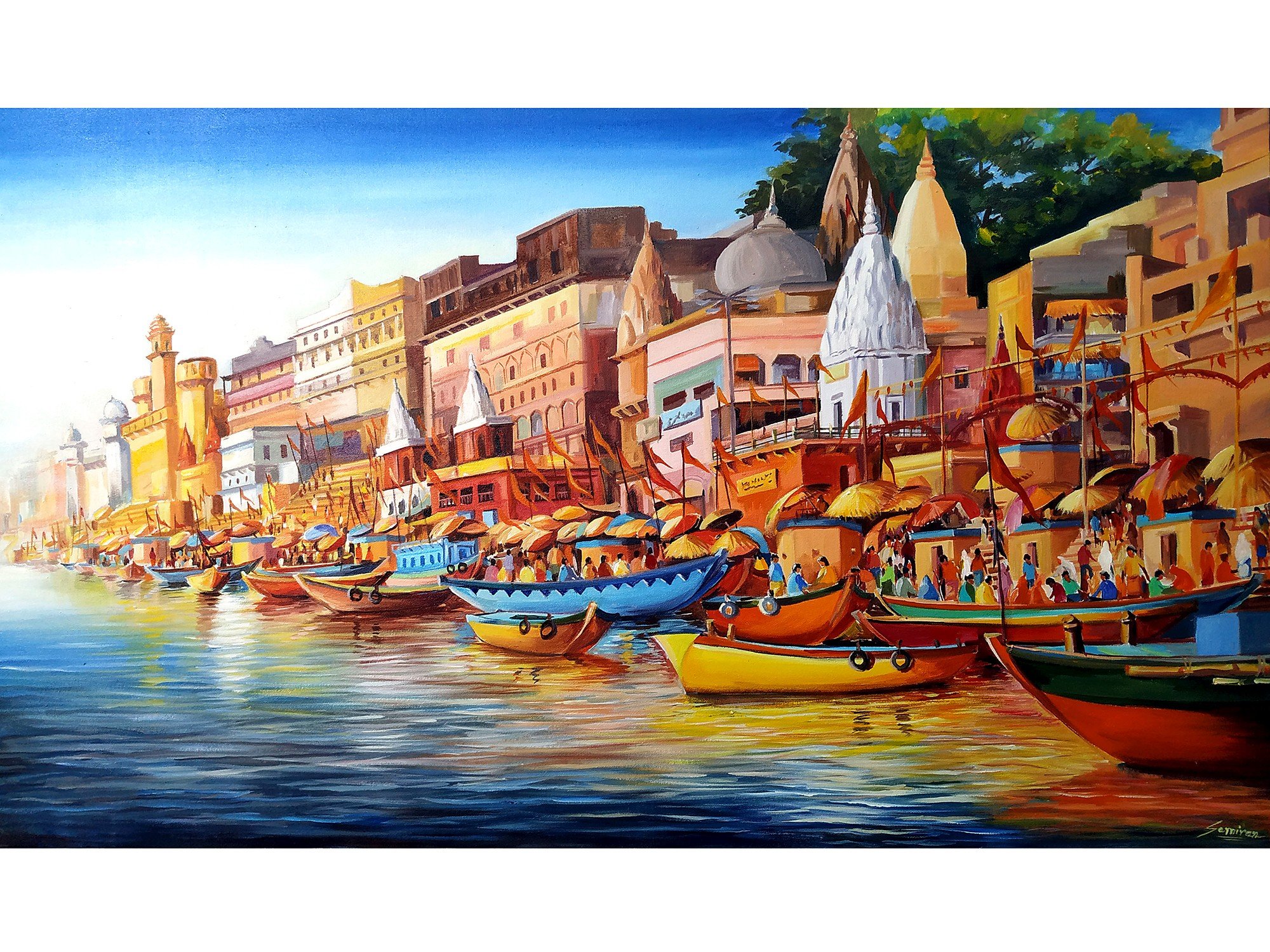This is a rectangular painting, approximately six inches wide by three inches high, depicting a vibrant coastal town by a body of water. The water, found in the lower portion of the scene, features blue waves with white ripples. Numerous colorful long, narrow boats, including yellows, oranges, reds, blues, and browns, are docked along a pier, populated with small figures whose colorful clothing and dark hair suggest a lively atmosphere. Some of the boats are equipped with umbrellas, providing respite from the sun.

Above the docks, a diverse crowd mingles on a boardwalk that stretches before an array of ancient stone buildings, some cylindrical with turrets in vivid colors like blue and yellow, and others with flat rooftops and intricate architectural details. Noteworthy among these is a circular yellow building, possibly a cathedral, adorned with statues on its arching top and accessed by stairs from the boardwalk. The buildings range from two to five stories and together create a multi-colored mosaic of yellows, browns, whites, and reds, giving a picturesque view of the town’s dynamic façade.

A long row of fluttering orange pennant banners extends from the left to the right of the image, contributing to the festive ambiance. In the background, the scene is framed by a blue sky on the upper left and a large green tree on the upper right, providing a natural contrast to the man-made structures. The detailed signature of the artist is visible in the bottom right-hand corner, adding a personal touch to this captivating portrayal of coastal life.